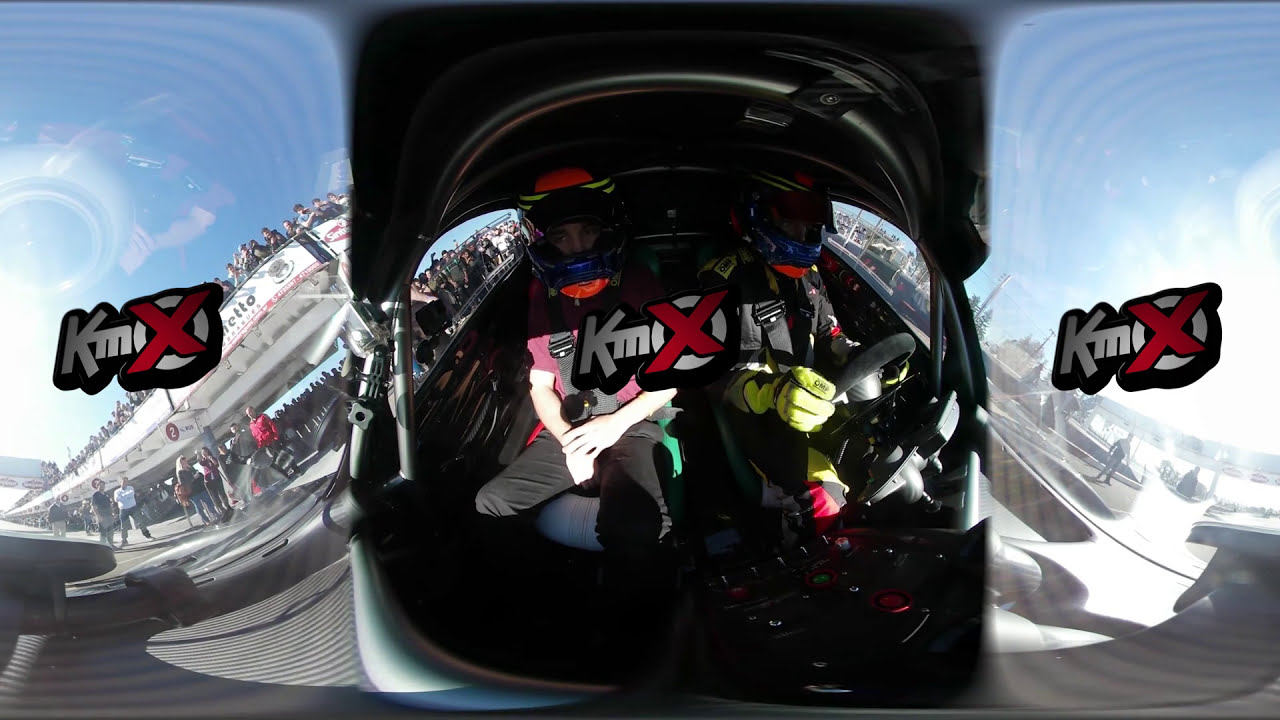The image displays a highly detailed 360-degree panoramic view from inside the cockpit of a racing vehicle, occupied by two individuals. Both are equipped with helmets featuring red and yellow detailing. The driver on the right is clad in a black top and yellow driving gloves, while the passenger on the left is dressed in a race jacket and black pants. The cockpit interior is predominantly black, with a central steering wheel and a dashboard visible. The fisheye lens effect notably warps the image, enlarging the occupants and distorting the surroundings.

Beyond the individuals, the panoramic view captures a bright, sunlit sky with bleachers and crowds of spectators forming two prominent rows, giving a vibrant, event-like atmosphere. There are also visible stands and people alongside the road. Adorning both sides of the image are the letters "KMX," stylized with an "X" through the "O," adding a recurring theme across the scene. Due to the intense sunlight, some image areas are washed out, reducing detail visibility and enhancing the panoramic distortion effect, making it challenging to discern specific elements clearly.